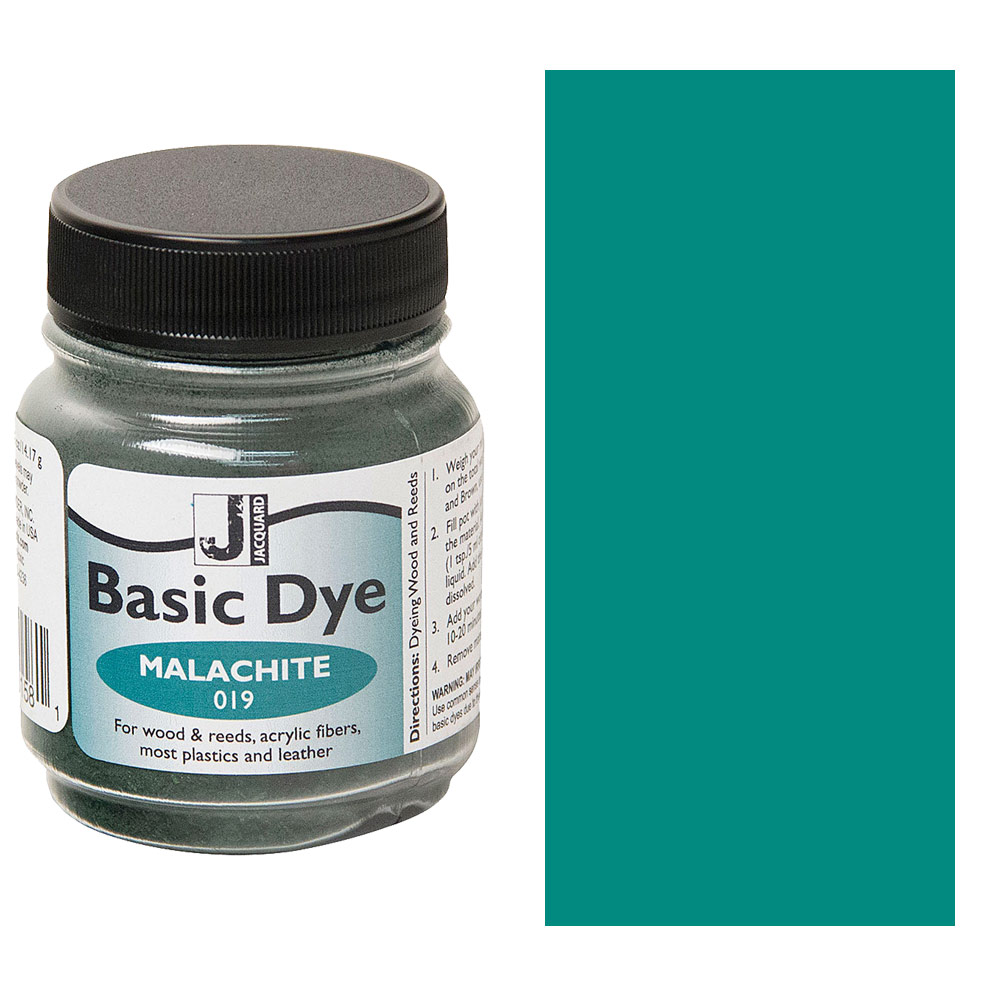A promotional photograph showcases a small, clear jar with a black screw-on lid, prominently labeled as "Basic Dye." The label, which features a white background with black text, includes the name "Malachite 019" in a blue oval. This dye is specified for use on wood and reeds, acrylic fibers, most plastics, and leather, suggesting its versatility for various crafting and artistic projects. To the jar's right side, a tall rectangular patch displays the dye’s resultant color—a darker greenish-blue hue. The jar itself contains a visible amount of the dye, although its exact color appears darker, more like charcoal or dark gray. Additional text on the label's sides is present but not legible in the photograph.